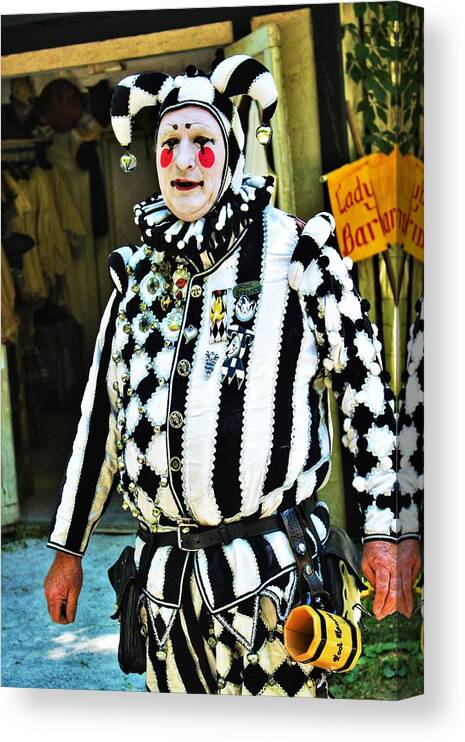The image captures a man dressed as a court jester, standing on what appears to be a rock driveway in front of an open structure with clothing draped on its sides. His entire outfit is an elaborate black-and-white ensemble, featuring both striped and checkered patterns. A traditional jester's hat with bells at each end adorns his head. His face is painted pale white, accentuated by thin, pronounced black eyebrows and surrounded by black paint with striking red circles beneath his eyes. His lips are also painted black. The jester wears a ruffled frill around his neck that matches his black-and-white motif. His shirt is ornate, adorned with medals, buttons, and bells running from top to bottom, all held together by a black belt that also carries leather sacks and a mug, suggesting he might collect tips. The belt cinches his outfit, seamlessly connecting to his matching pants. His hands appear old and liver-spotted. In the background, a sign reading "Lady Baron" in yellow can be seen, hinting at a possible renaissance fair setting.